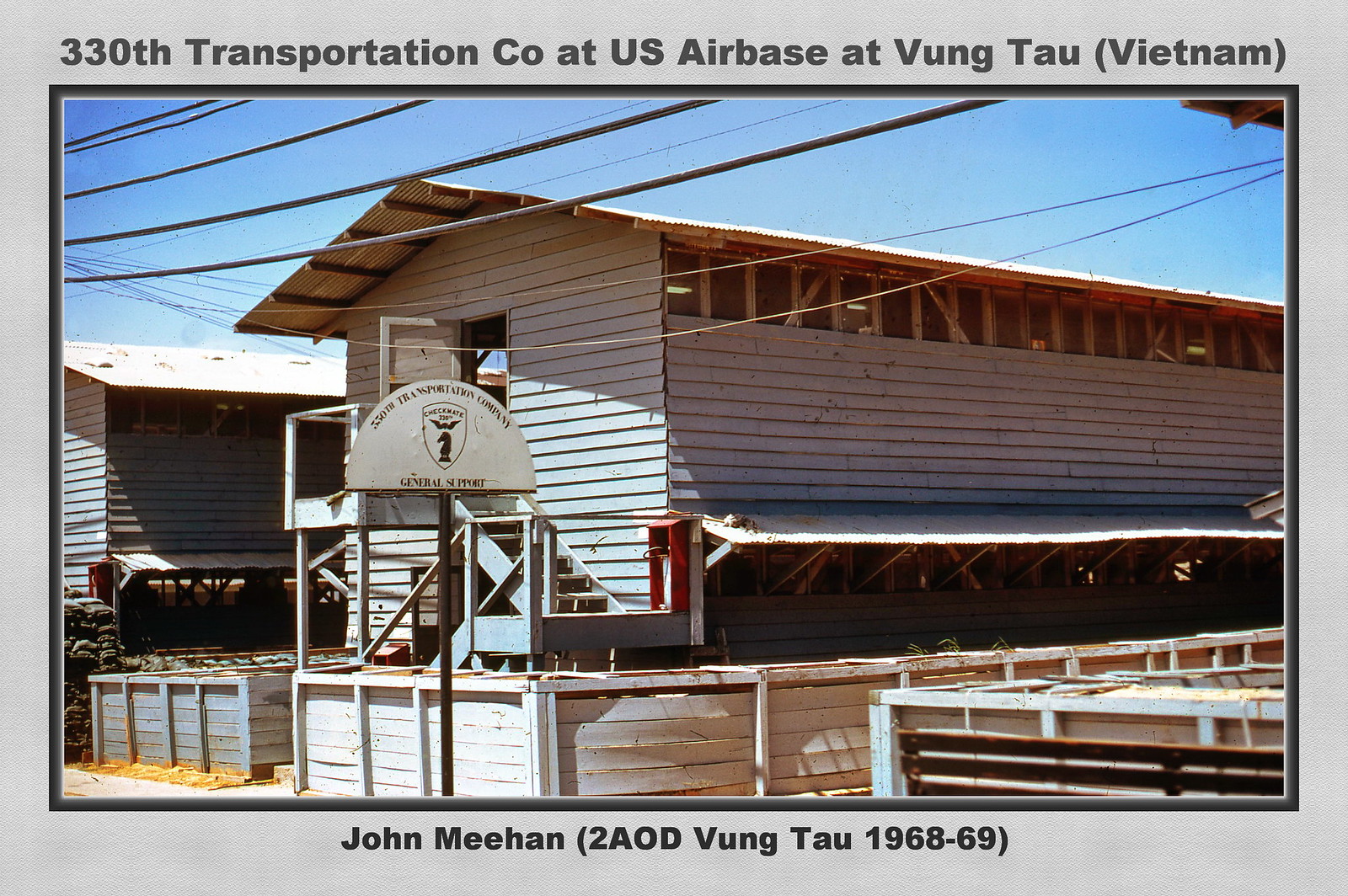This photograph depicts a large white building located at the U.S. Air Base in Vung Tau, Vietnam. The building, made of white wooden slabs, features a triangular roof and appears to be one of a series of identical structures. Adjacent to it, another building of the same design can be seen, suggesting a row of similar buildings. A prominent sign in front of the building reads "330th Transportation Company, General Support." The sign includes a shield logo with the word "Checkmate" inscribed on it. Above the photograph, a gray border contains the text "330th Transportation Co. at U.S. Air Base at Vung Tau, Vietnam." At the bottom, the same gray border lists "John Meehan, 2AOD, Vung Tau, 1968-69." The background shows a blue sky with power lines running across.